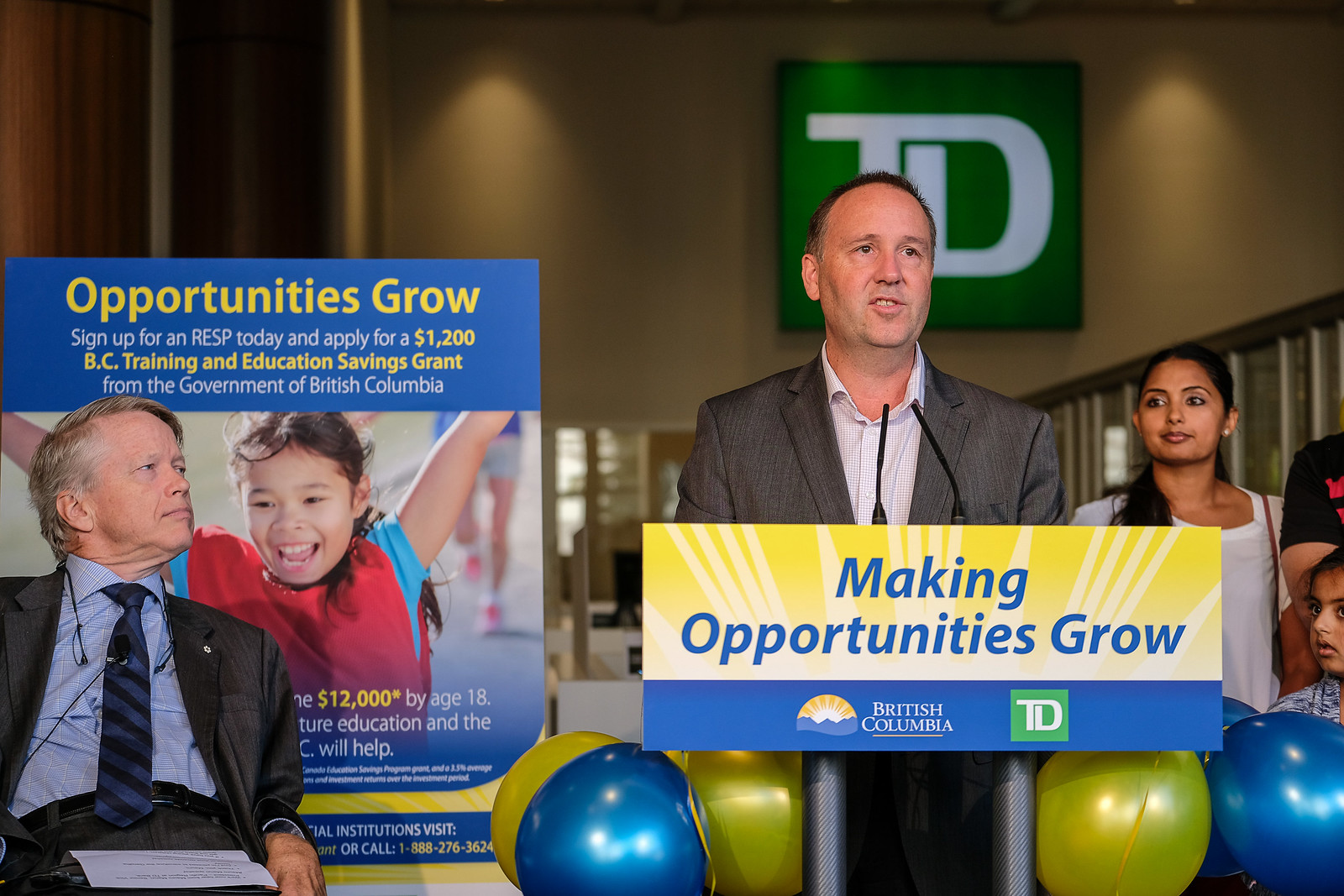In this photograph, a middle-aged man is delivering a speech while standing at a podium, adorned with a bright yellow and blue sign that reads "Making Opportunities Grow" and "British Columbia" beneath it. The podium also has balloons attached below it and is positioned in front of a backdrop featuring the TD Bank logo in green and white text. Behind him is a staircase and wall. To his left, there's a man in a suit, possibly sitting in a wheelchair, watching him intently. To his right is a woman in a white shirt, also looking up at him, along with some children situated further right. Additionally, there’s a large poster to his left depicting a child with raised arms, emphasizing the theme "Opportunities Grow."